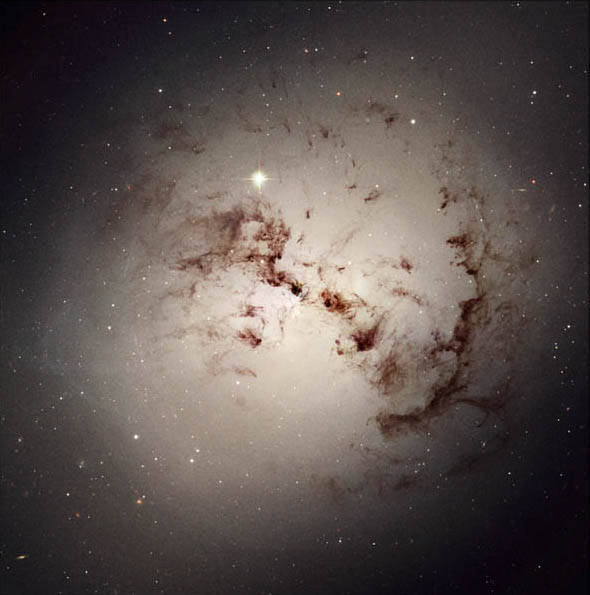The image depicts a galaxy-themed scene set in outer space. The bottom right-hand corner starts as an inky black, gradually transitioning to a soft gray. Brown streaks begin to emerge from this gray section, adding texture and depth. On the bottom left side, the image starts with a gray hue that spans the entire lower portion of the picture. This gray transitions into a light purple, forming a circular shape in the center. This purple circle is interspersed with brown streaks, adding a dynamic contrast. A brilliant white light glows at the top of the scene, surrounded by numerous white specks that mimic stars, illuminating the galaxy. The top left and right corners of the image also feature a black background, framing the celestial composition beautifully.